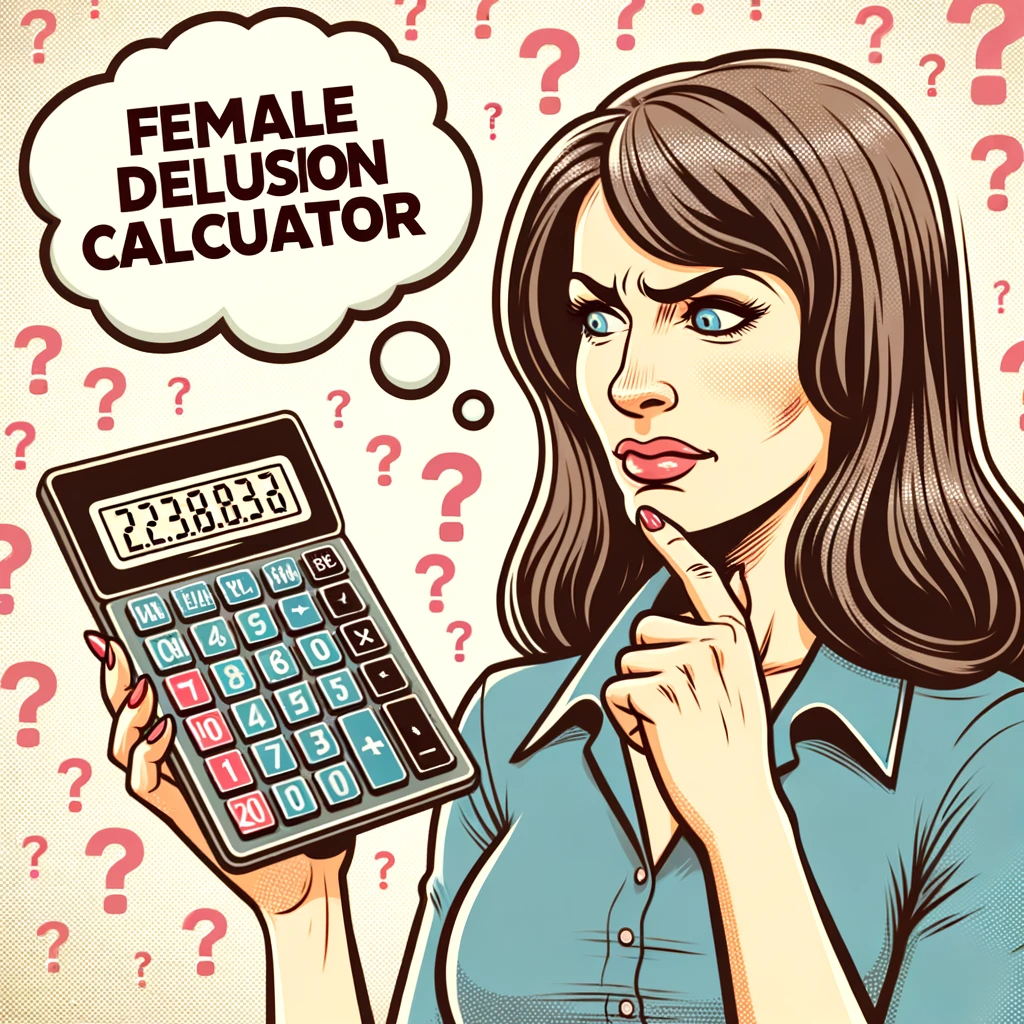In this vibrant color illustration, a woman with long, brown hair cascading down to her shoulders is depicted against a white background adorned with numerous red question marks. Her striking blue eyes stand out, complemented by pink lipstick. She is wearing a turquoise button-down collared shirt, adding a touch of color to her appearance. The woman’s left index finger is thoughtfully placed on her chin, with the remaining fingers of that hand curled inward. In her other hand, she holds a calculator displaying the sequence 2.2.3.8.8.3.8. The expression on her face is one of concern or confusion, as she frowns while looking at the calculator. To the left of her head, a thought bubble emerges with the text "Female Delusion Calculator," indicating her contemplation.